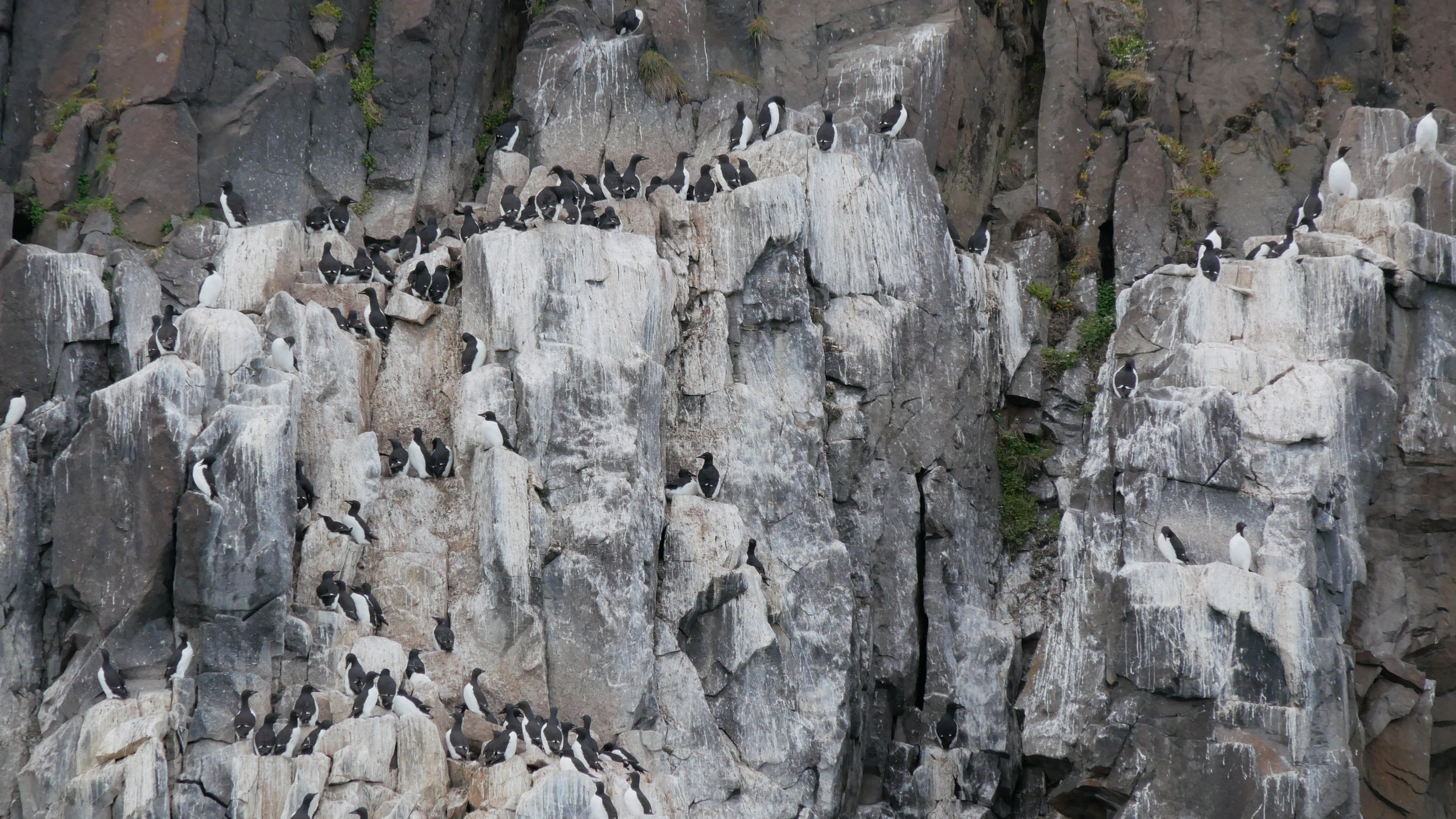This photograph, likely taken in the Antarctic, captures a dramatic cliffside teeming with penguins. The cliff, composed of white, gray, and brown rocks, showcases green vegetation sprouting from its crevices alongside white streaks that hint at the frequent presence of the birds. Penguins, easily identified by their black and white "tuxedo" appearance, are scattered across the face of the cliff. Clusters of these birds are concentrated in the bottom left and the top center-left of the image, while solitary figures are perched on individual outcrops. The shot, seemingly taken from a distance, offers a sweeping view of hundreds of penguins in various positions - some standing, others sitting - on the rocky precipice. The interplay of natural colors and the animated presence of the penguins creates a captivating scene.